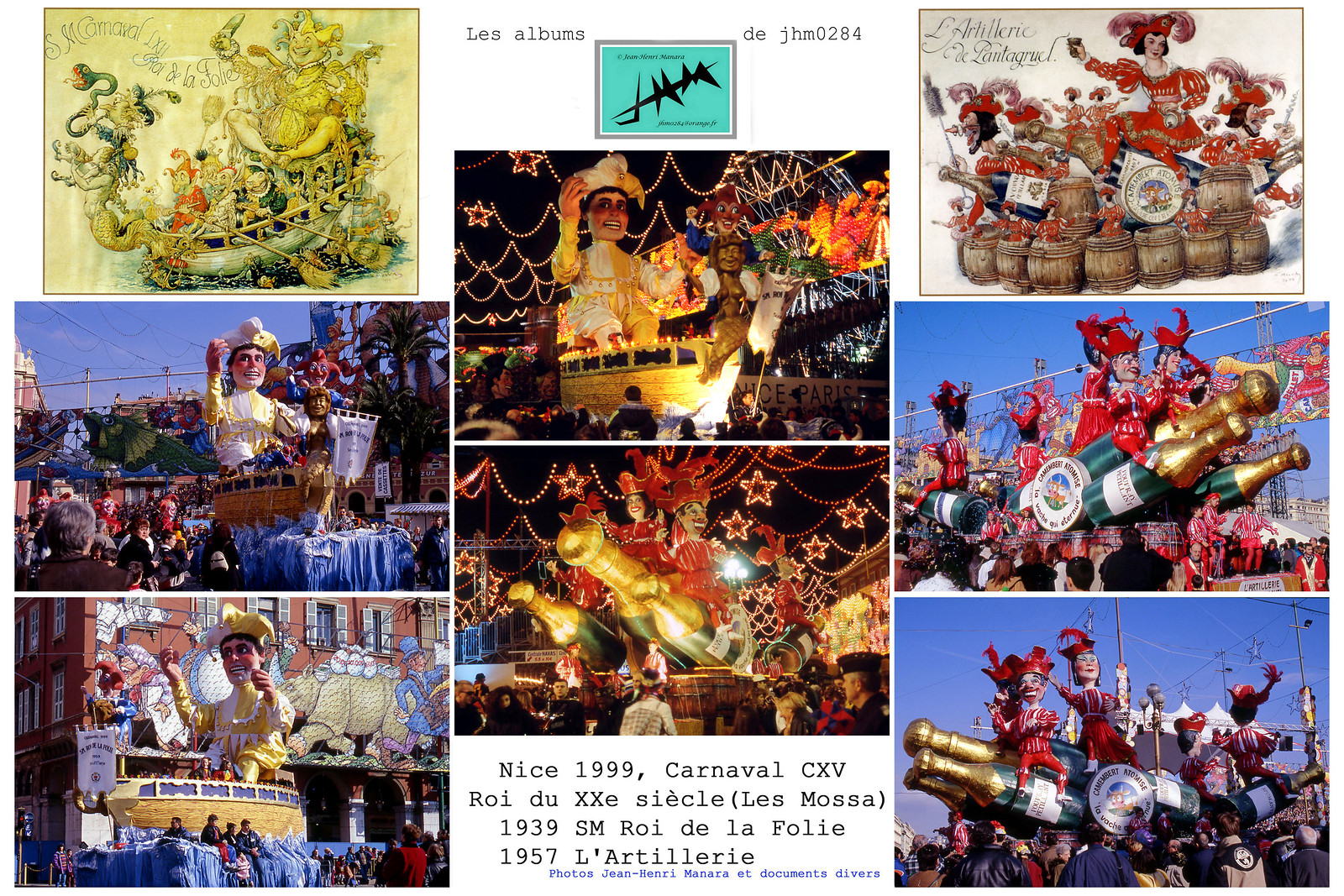The image is a vibrant collage featuring eight distinct photographs that present a Mardi Gras-themed festival. There are three photos on the left, three on the right, and two in the center. The overall scene is lively, with spectators surrounding the elaborate and colorful floats. The top left picture has a slight yellow and white tint and possibly an older, more antique feel. Below it are additional images of the floats. On the top right, there's an image of a person atop barrels, dressed in red, with two subsequent pictures depicting the related float just beneath.

The central photos display similar floats with text overhead that reads "Les Albums de J.H.M. 0284," along with a blue logo labeled "J.M.M." Below these central images, inscriptions are in French: "Nice 1999, Carnival CXV, Radu XXE, and then SIECLE Le Massa, 1939 S.M. Roy de la Foly,” and “1957 La Thillerie.” Each frame reveals extravagant floats and cheerful crowds in an outdoor setting under clear blue skies.

Among the decorated floats, noted features include a man riding a boat and others on enormous champagne bottles. The photographs capture the vibrant essence of the parade, filled with detailed and colorful designs, demonstrating the ornamental floats and jubilant atmosphere of the celebration. Additionally, the mention of Jean-Henri Mahara and various documents suggests a rich historical context and preservation of past festive moments.